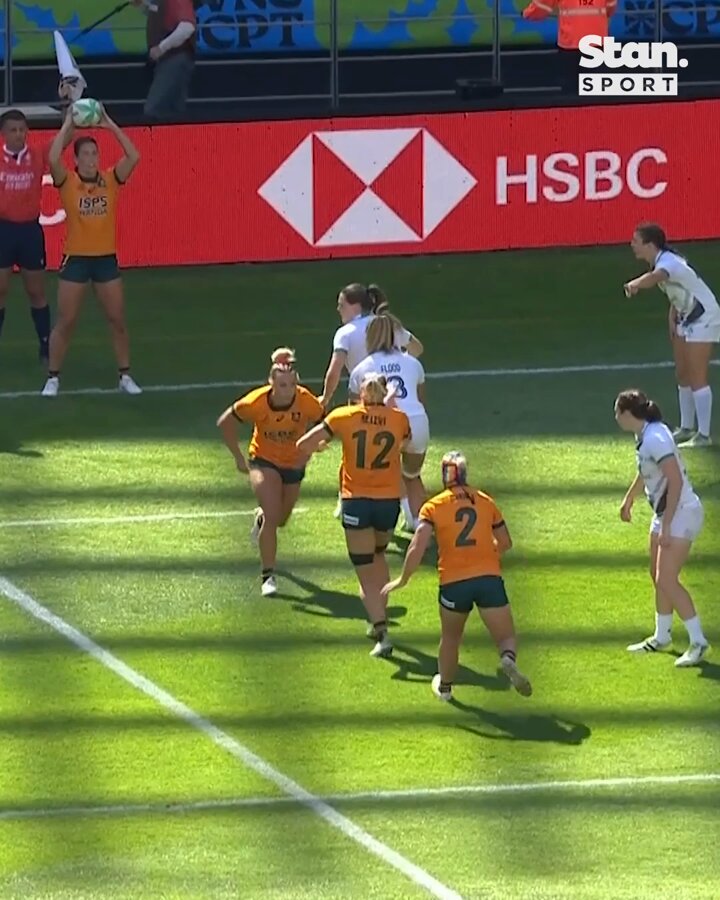This action-packed photo captures a girls' soccer game under the bright sun, with shadows stretching across the grassy field. At the top right corner of the image, "Stan. Sport" is displayed prominently. The backdrop features a large red banner with "HSBC" in bold white letters. The scene on the lively green pitch is divided between two teams—one in vibrant orange uniforms with black shorts and the other in all-white uniforms. 

To the top left, a young woman in an orange jersey is about to throw the ball back into play, holding it high above her head. Next to her stands a referee in a red shirt and black shorts. Behind them, elevated above the field, two individuals are walking on a platform; one is partly visible in an orange jacket, and the other, only partially visible in a red shirt. 

On the field, three women in orange are actively running: one is headed towards the left, another just ahead of her, and the third running towards the camera. Meanwhile, the team in white is strategically positioned in a triangle formation on the right side of the photo, ready to intercept the play. The vibrant energy of the game is palpable, capturing a moment of fierce competition and teamwork.